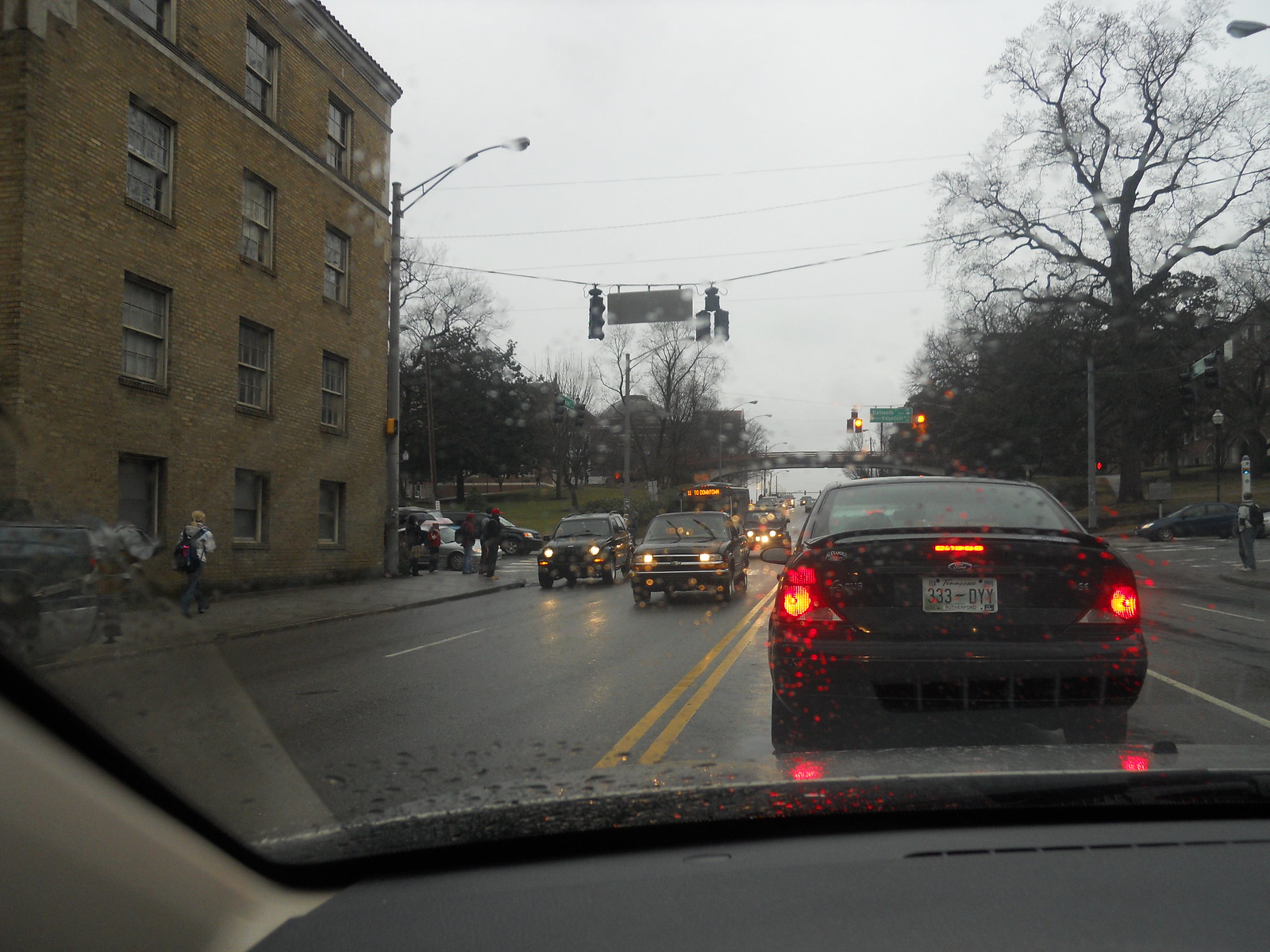A photograph captures a rainy street scene as viewed from the driver's seat of a vehicle. Directly ahead is a black sedan with its brake lights glowing, halted before a traffic light that is transitioning to yellow. The windshield is speckled with raindrops, suggesting a recent or ongoing shower. In the adjacent lane, a black Jeep and a black pickup truck navigate through the wet double-lane traffic. To the left, a four-story building constructed of tan brick stands prominently, with a handful of pedestrians gathered on the sidewalk, waiting to cross the street. The setting is a bustling four-way intersection, with additional pedestrians visible on the right corner, poised to traverse several lanes of oncoming traffic.